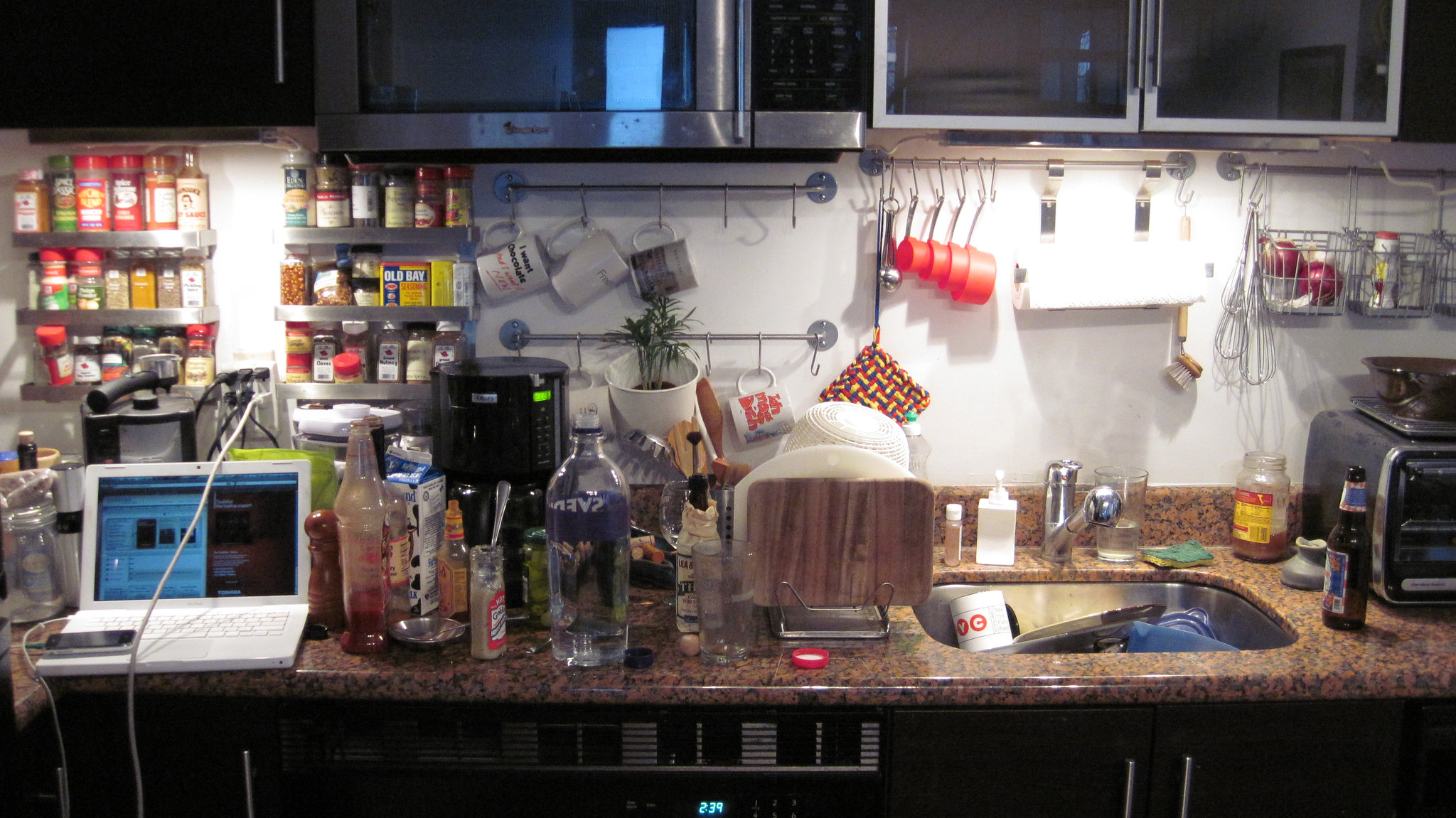A well-stocked kitchen bustling with activity stretches across the frame. On the upper left, a metal shelf cradles an assortment of colorful spices, including a distinctive yellow jar with a red cap of Old Bay seasoning. These spice containers range in materials from glass to plastic, all illuminated by a soft, warm light. 

At the bottom left, an open laptop sits with a cell phone charging on top of it, connected to an outlet by a tangle of cables. Below this setup, a sleek dishwasher is discernible by its display and ventilation slots. Spanning across a speckled brown and black granite countertop are numerous bottles, including a clear one that looks like it contains vodka, and various sauces and ingredients with labels that are difficult to read clearly.

In the background, a black cylindrical coffee maker stands ready, accompanied by a white pot hanging from a silver hook. Several mugs dangle from the same row of hooks. On the upper right, a silver bar holds red measuring cups, and at the very top, silver containers filled with vegetables like onions are visible, along with a packaged item. 

Near the center of the countertop is a drying rack with a wooden cutting board nestled inside, alongside an array of white items. Off to the right, a shiny silver faucet presides over an overflowing sink. Adjacent to the sink, an open beer bottle and a jar containing a bit of brown liquid sit, next to a microwave. The scene captures a moment in a vibrant, lived-in kitchen, rich with culinary possibilities.